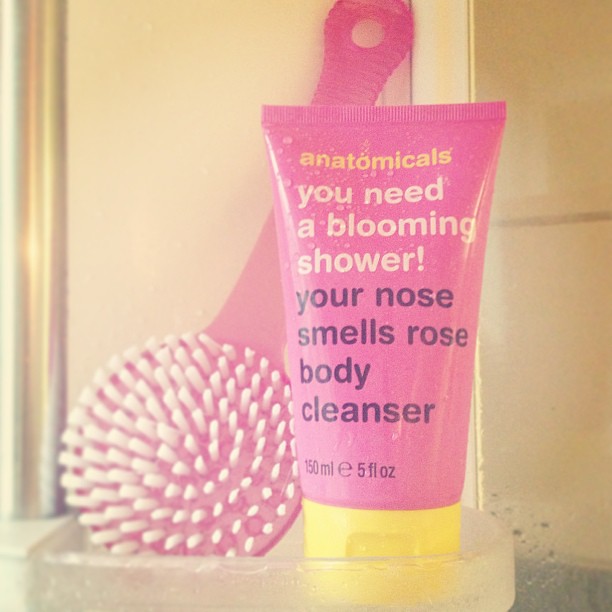The image depicts a bathroom setting with a pink tube of body cleanser and a matching pink-handled brush. The tube stands on its yellow cap and prominently features the brand "anatomicals" in yellow text, followed by the phrases "You need a blooming shower" in white and "your nose smells rose body cleanser" in black. The text also mentions the volume as "150 ml, E 5 FL ounce." The brush, with its circular head and white bristles, rests alongside the tube within a clear plastic container. The background reveals yellowish-tan wall tiles and small water droplets, indicative of a steamy shower environment.